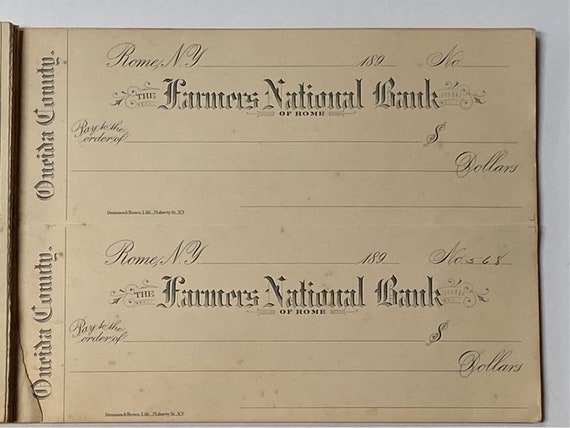This photograph features a pair of blank checks from the 1800s, specifically issued by the Farmers National Bank of Rome. The checks, which are a parchment beige color and show signs of aging with a weathered and yellowed appearance, are stacked one on top of the other. Each check is meticulously designed with "Rome, New York" written in the top left, followed by a space for the date marked with "18-9" where the user can fill in the remaining two digits. Additionally, there is space for the check number, with "568" visible on the top check.

The bank's name, "The Farmers National Bank of Rome," is elegantly scripted underneath the date. There are printed prompts for "pay to the order of," followed by a blank line, a dollar sign, another blank line for the amount in words, and a final blank for the signature. Oneida County is printed vertically on the left side of the checks, adding a historical touch. The format of these checks suggests they were part of an old checkbook, with indications of perforations where they could be torn out after being filled in and signed.